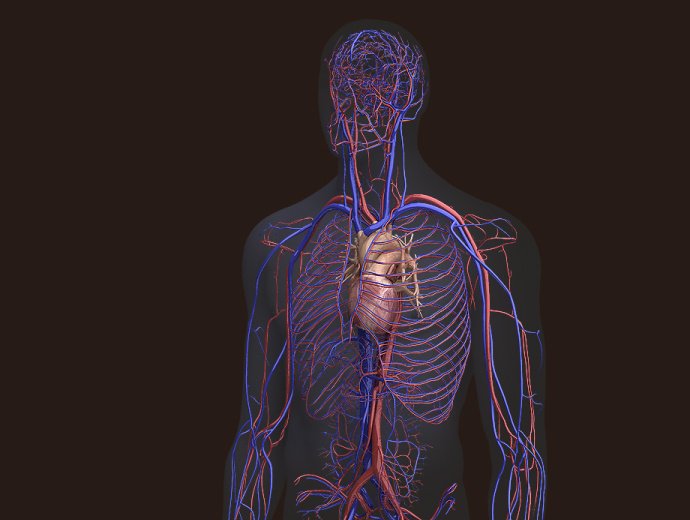The image is a detailed anatomical drawing of a human cardiovascular system set against a completely black background. The figure shows a transparent, grayish outline of a human body, allowing the vivid depiction of the cardiovascular components within. The body's intricate network of red arteries and blue veins is prominently featured, running throughout the torso, arms, and head. The heart, central and depicted in a brown hue, sits in the middle of the chest with two purple lungs flanking it. These veins and arteries are depicted with striking clarity, extending from the heart to the far reaches of the body, including the torso and arms, and even up to the brain, where a dense cluster of smaller blood vessels can be seen. Overall, the diagram provides a comprehensive view of the human cardiovascular system with a stark, black background enhancing its anatomical precision and detail.